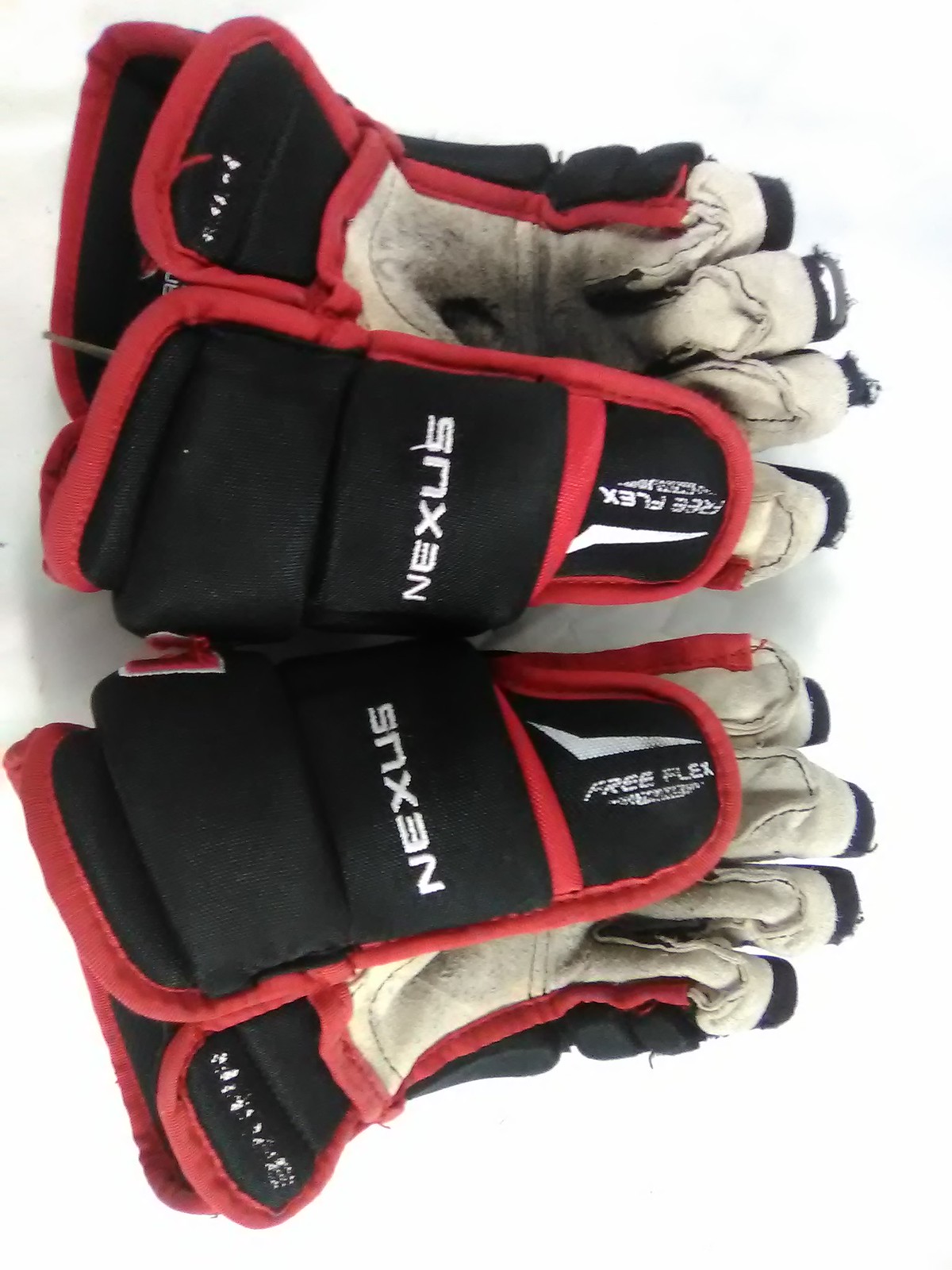The image depicts a slightly overused pair of hockey gloves, positioned horizontally with their palms facing upwards. The gloves are oriented such that the finger tips are on the right side of the image while the cuffs are on the left. The gloves feature a predominantly black exterior with red outlines, and the inner palm area is white or off-white in color. The thumbs of the gloves are facing each other and are marked with white lettering; on the thumb portion it reads "Nexus," and on the thumb tips the text reads "Free Flex," accompanied by a boomerang-like white logo. The fabric at the top of the gloves is slightly frayed, and the very bottom shows some white lettering that is also frayed. The background of the image is white, and the gloves appear to be side by side, emphasizing their wear and tear.